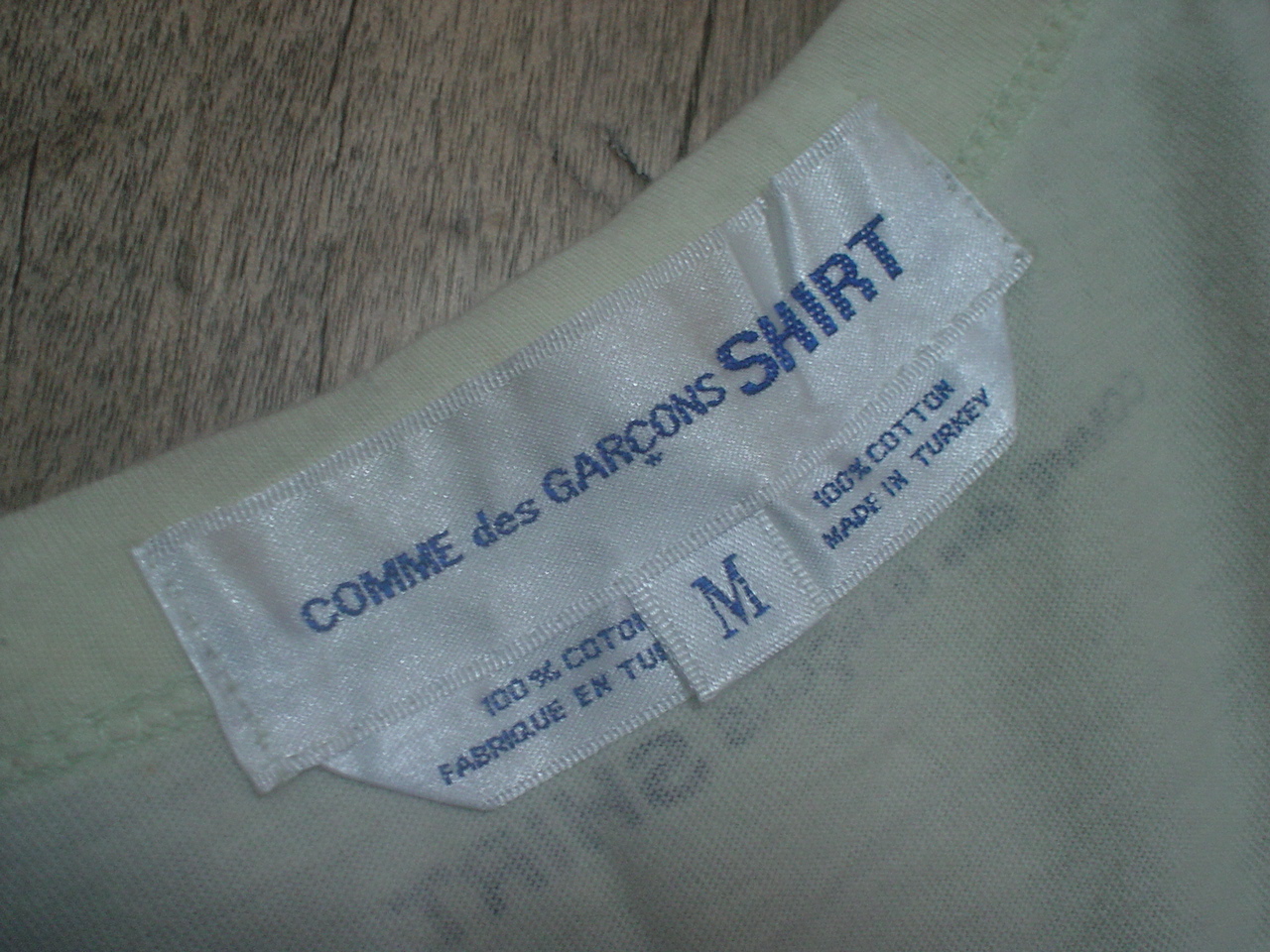Foregrounding an off-white shirt, this image features a prominent white tag displaying text in a foreign language, likely identifying the product or its maker. The tag reads "Comme des Garçons Shirt" with "Comme des Garçons" in smaller, capital letters and "Shirt" in larger, capital letters. The "C" in "Garçons" includes a distinctive squiggly line underneath it, indicating its French origin. The text on the tag is predominantly blue, except for "D-E-S," which stands out in a different color. Additionally, the tag specifies that the shirt is made of 100% cotton, with a note about its fabrication in a presumably foreign language, featuring "T-U" followed by a capital "M" encased in a box. To the lower right, the tag confirms it is made in Turkey. The shirt rests on what appears to be varnished wood, visible in the upper left-hand corner of the image, enhancing the overall aesthetic.